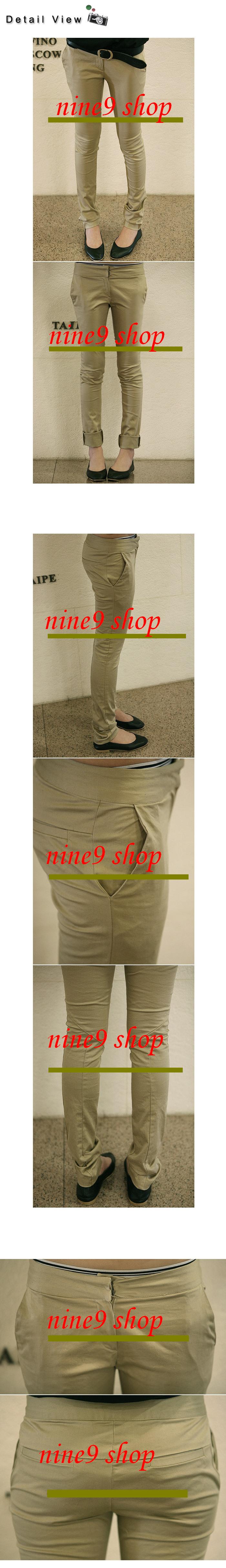This image features a vertically arranged strip of seven sectional photographs showcasing a woman modeling tight-fitting, legging-style pants. The photos are organized in three distinct sections: at the top, two rectangular images display the woman facing forward, highlighting the front of the brown pants and her feet slightly pigeon-toed in black flats. Red text is centered on these top images. The midsection comprises three images, presenting a side view, a back view, and a detailed close-up of the pants' back pocket area. These images also feature red text, with a hint of a yellow line behind it. The bottom section consists of two horizontally aligned images that zoom in on the back area and fit of the pants. The woman, set against a light-colored wall and medium gray carpet, wears a black top and a belt with the pants, providing a comprehensive view from multiple angles including side, back, front, and various close-ups.